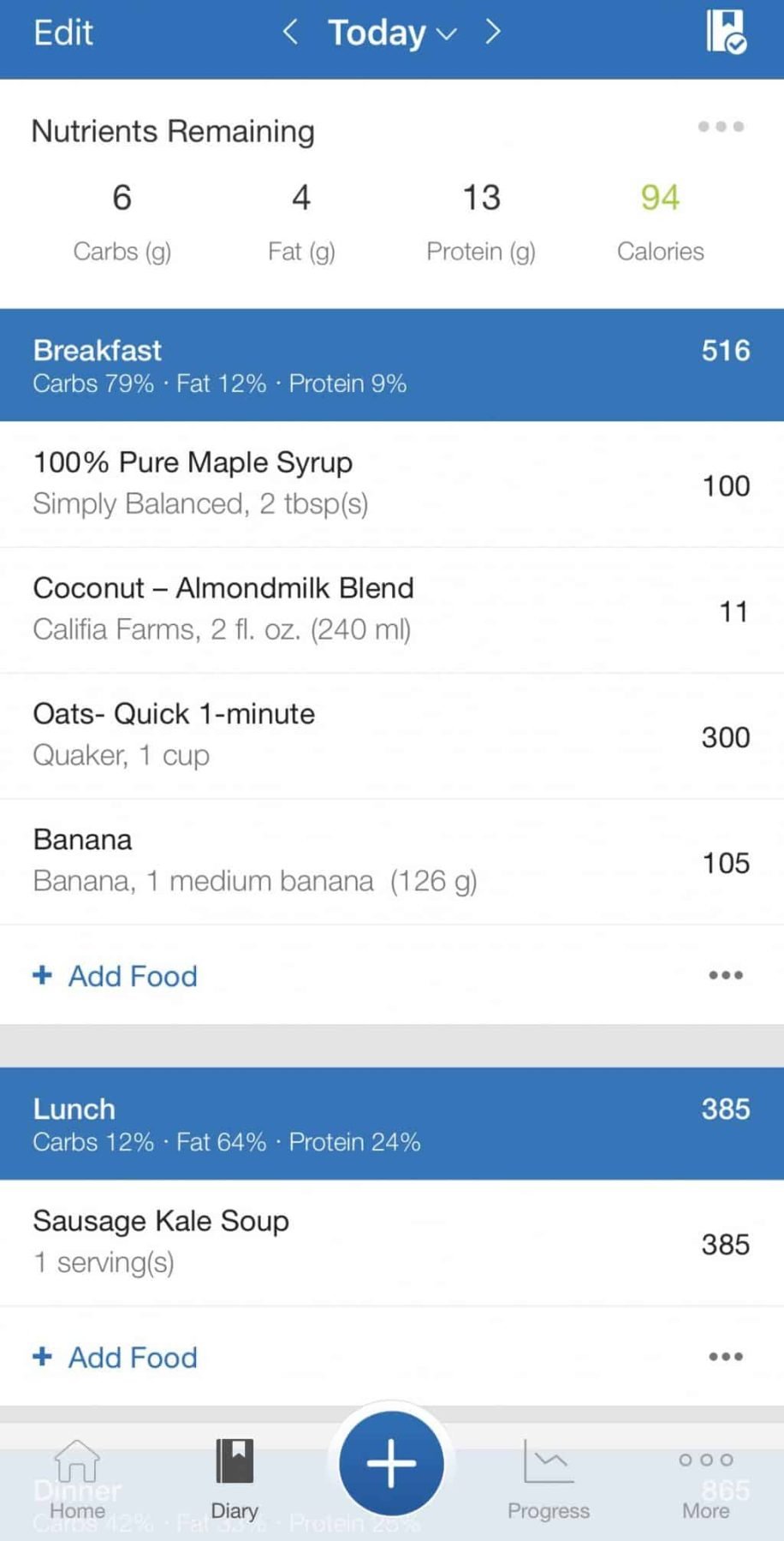In the image, there is a detailed screenshot from a nutrition tracking app displayed on a smartphone. At the very top of the app, there is a blue navigation bar containing the options "Edit," symbols for navigation with a less-than and greater-than sign, a dropdown menu labeled "Today," and a book icon with a checkmark next to it—all in white text.

Underneath this navigation bar, there's a section titled "Nutrients Remaining," detailed as follows: 6 grams of carbohydrates, 4 grams of fat, 13 grams of protein, and 94 calories. The text for the macronutrients and calories is rendered in black, while the numerical value "94" is highlighted in a golden color.

The screenshot further breaks down the diet into distinct meal sections, all with blue headers and white text. The first section labeled "Breakfast" indicates a caloric intake of 516 calories, distributed as 79% carbs, 12% fat, and 9% protein. The detailed food items include:
- 100% Pure Maple Syrup, Simply Balanced, 2 tablespoons (100 calories)
- Coconut Milk Almond Milk Blend, Califia Farms, 2 fluid ounces (240 milliliters, 11 calories)
- Quick One Minute Oats, Quaker, 1 cup (300 calories)
- A medium banana, 126 grams (105 calories)

Following the food details, there is a blue plus sign and the "Add Food" button, alongside an ellipsis indicating more options.

The next blue section labeled "Lunch" shows a total of 385 calories, with percentages of nutrients as 12% carbs, 64% fat, and 24% protein. This section details:
- Sausage Kale Soup, 1 serving (385 calories) 

Again, there’s a blue "Add Food" button at the end of this section.

Along the bottom of the app interface, there is a navigation bar featuring icons and labels in white: "Home" with a house icon, "Diary" with a book icon, "Progress" with a line graph icon, and "More" with an ellipsis. In the center of this bar, there is a prominent blue circle with a white cross, likely for adding new entries. 

The color scheme demonstrates a well-organized interface with blue tones for headers and important buttons, black for food items, and golden highlights showing significant values.